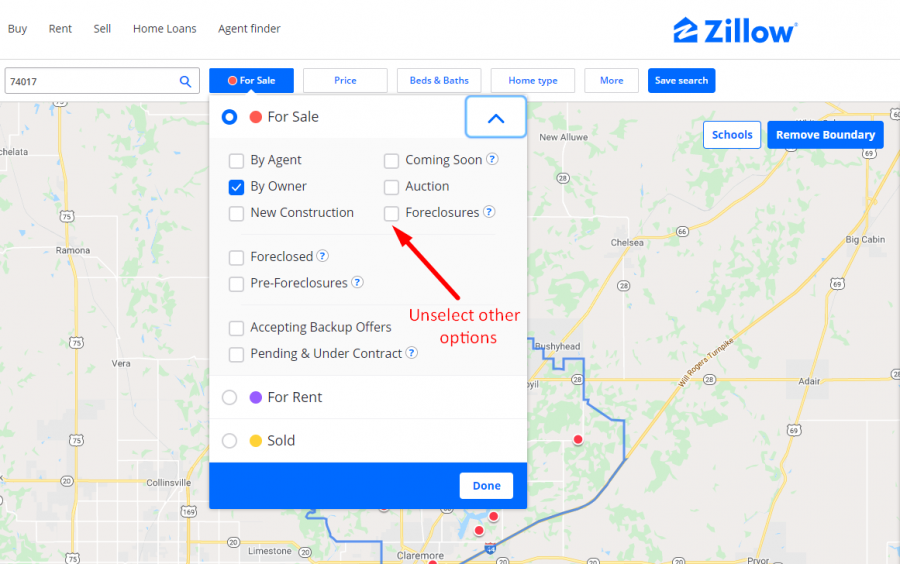The image showcases an interactive map interface on the Zillow website. Prominently displayed at the top right corner is the Zillow business name, accompanied by its distinctive logo on the left. The map itself is detailed with several overlays and interactive options. Key navigation links such as "Buy," "Rent," "Sell," "Home Loans," and "Agent Finder" are clearly visible. Various interactive filters are also present on the map, including options for "For Sale," "Price," "Home Type," "More," and "Save Search," among others.

Additionally, there are several specific real estate categories detailed, such as "By Owner," "New Construction," "By Agent," "Coming Soon," "Auction," "Foreclosures," "Foreclosed," and "Pre-Foreclosures." These options suggest the wide range of real estate activities and listings that can be explored.

In the background, the map highlights several locations including Vera, Ramona, New Alley, Big Cabin, Chelsea, and Adele. These geographical markers provide context for the areas being targeted or displayed on the Zillow interface. Overall, the image effectively conveys the comprehensive and user-friendly nature of Zillow's real estate listing and search platform.